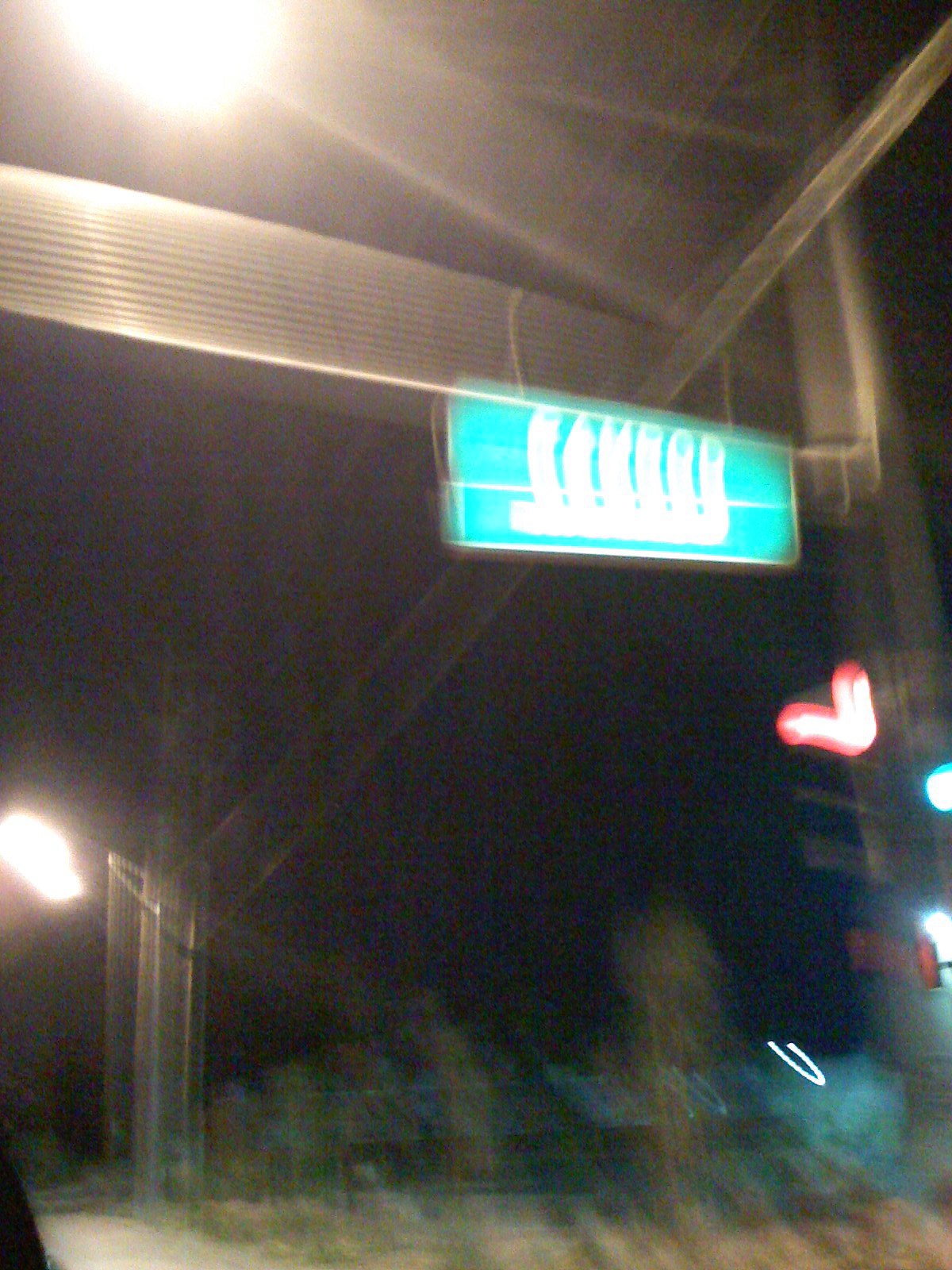This photograph captures an urban street scene, though the image is extremely blurry. It appears that the photographer was either in motion or accidentally dropped their camera or cell phone while taking the shot. On the right side of the frame, a stoplight is visible, displaying a green light. Above this, the image reveals a structure that looks like a metal bridge or metal posts designed to hold street signs and stoplights. In the background, there is a small line of trees, indicating a natural element amidst the urban setting. The top and middle sections of the photograph show a few lights, contributing to the city's illuminated atmosphere. Near the center-right of the image, a green rectangular street sign with white text is visible, though the text is illegible due to the blur.